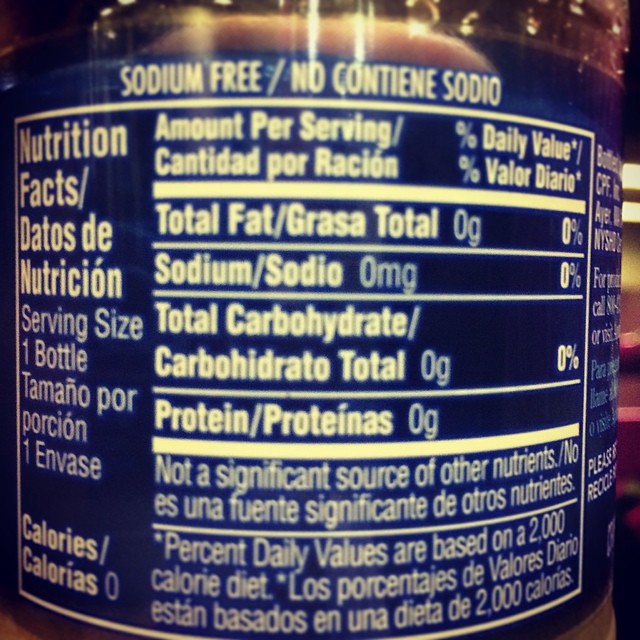Here is an elaborate and detailed caption for the given image:

"The image depicts a nutrition label from a bottle, characterized by its dark blue or black background with contrasting white and yellow text. Prominently displayed at the top of the label are the words 'Sodium Free,' followed by a similar declaration in another language. On the left side, the label begins with 'Nutrition Facts,' also translated into what appears to be Spanish. The serving size is listed as one bottle, accompanied by the information that the product contains zero calories. Detailed nutritional information is provided, including sections for 'Amount per Serving,' 'Total Fat,' 'Sodium,' 'Total Carbohydrate,' and 'Protein.' A statement at the bottom clarifies that the product is 'not a significant source of other nutrients.' Additionally, it notes that the percent daily values are based on a 2,000 calorie diet. Each English term on the label is immediately followed by its Spanish translation, ensuring bilingual accessibility."